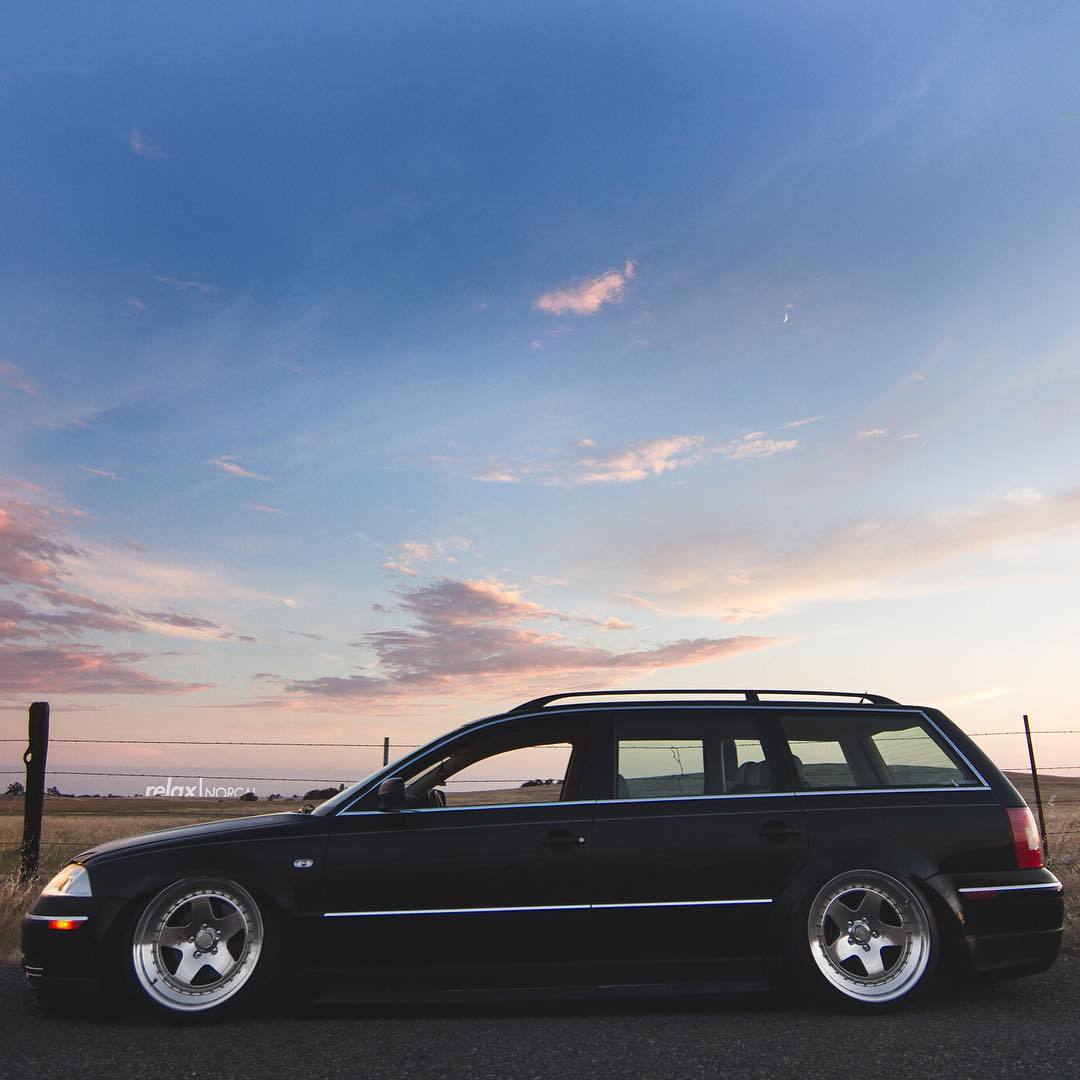The image captures a black station wagon with silver rims parked on the side of a dark concrete road, facing the left. The left side of the car is visible, showing yellow and white headlights and red taillights. Behind the car runs a dark-colored wire fence with wooden posts, separating it from a large grassy field. In the distance, the lush field is bordered by a line of trees. The sky above transitions from a deep blue at the top to a lighter blue, almost white at the horizon, featuring feathery cirrus clouds in shades of gray and white. There are also hints of pink near the bottom of the sky. In the rear of the car, barely legible white text appears to read "relax." The overall scene blends the serene, natural backdrop with a touch of the functional urban environment, typified by the station wagon and its setting. The model and year of the car suggest it might be from the 90s, not too old but not modern either.